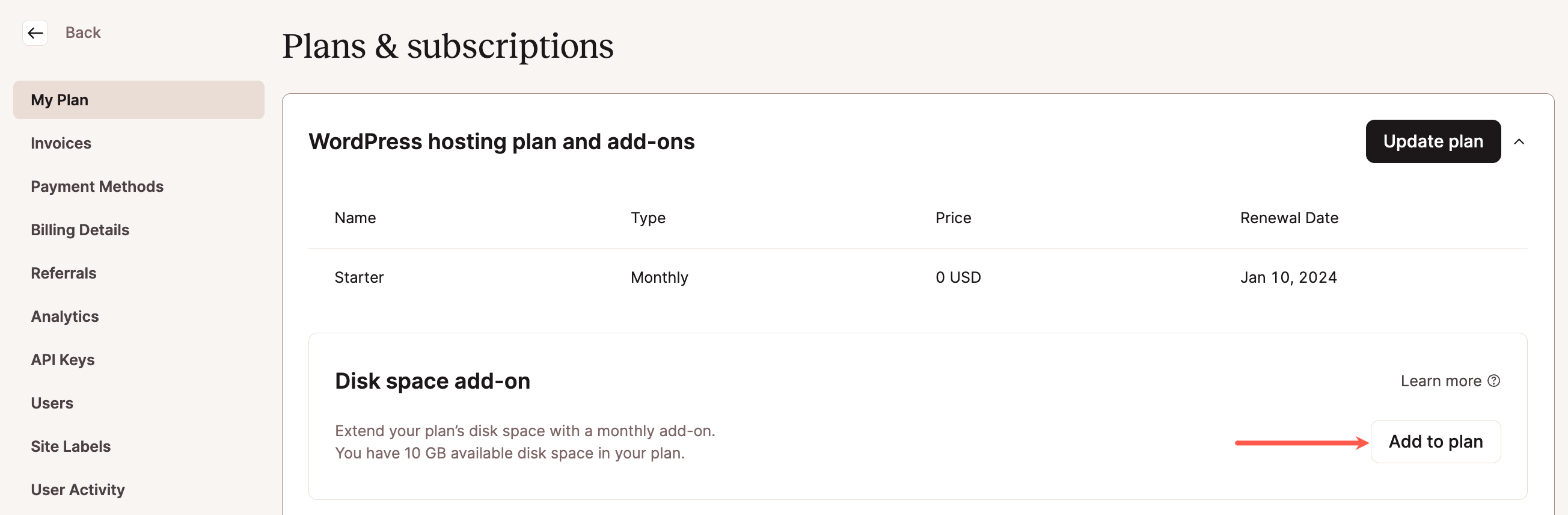The image captures a screenshot of a computer screen displaying a user interface related to plans and subscriptions. The predominant background color is a very light beige, providing a neutral and clean aesthetic. At the top-left corner, the title "Plans and Subscriptions" is prominently written in black.

Below the main title, a vertical menu on the left side lists various options in the beige area, including "My Plan," "Invoices," "Payment Methods," "Billing Details," "Referrals," "Analytics," "API Keys," "Users," "Site Labels," and "User Activity."

At the very top of this beige area, there is a back button located within a lighter beige square, with the word "Back" clearly indicated for easy navigation.

Moving down the screen, a large white rectangle stands out, labeled "WordPress Hosting Plan and Add-ons." This section is organized with headers for "Name," "Type," "Price," and "Renewal Date." Underneath these headers, the following information is presented:
- Name: Starter
- Type: Monthly
- Price: 0 USD
- Renewal Date: January 10th, 2024

Additionally, a black button labeled "Update Plan" is positioned at the top, offering the user an option to modify their current subscription plan. The overall layout is clean and user-friendly, facilitating easy management of plans and subscriptions.